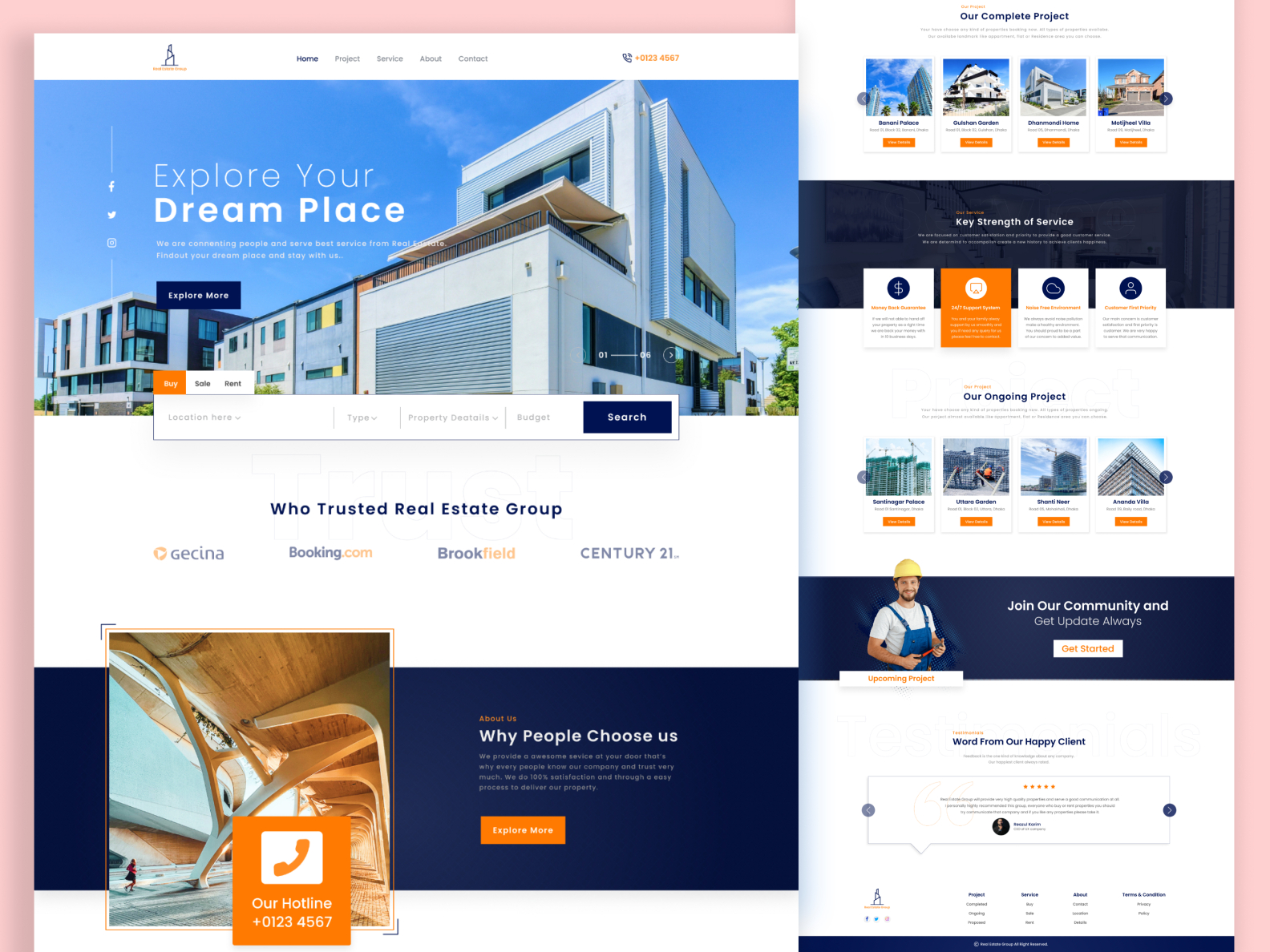This is a detailed caption for an image of a real estate group's web page:

The web page for a real estate group features a sophisticated design with a company logo situated in the upper left-hand corner. Although the company name text is small and difficult to read, it accompanies the logo icon. A white navigation ribbon spans the top of the page, including tabs labeled "Home," "Project," "Service," "About," and "Contact." On the far right edge of this ribbon, a phone icon with a red phone number is displayed prominently. Just below this section lies an image of several modern buildings, which appear to be upscale homes, as suggested by the tagline “Explore Your Dream Place.” The day depicted in the image is sunny with a bright blue sky, enhancing the modern, sleek architecture of the homes.

Social media icons for Facebook, X (formerly Twitter), and Instagram are available for easy connectivity. Beneath the image, users can choose between options marked "Buy," "Sale," or "Rent," followed by a search box for specific inquiries. Further down on a white background, the text in blue reads “Who Trusted Real Estate Group,” listing affiliated companies such as Justina, Booking.com, Brookfield, and Century 21.

On a navy blue background, the section titled “Why People Choose Us” in white text offers a brief explanation, alongside an orange box inviting users to explore further. Below this, another image showcases a modern architectural building with a young woman walking underneath an archway. Additionally, there is an orange box with a white inside and an orange phone icon, labeled “Our Hotline” in white text along with a contact phone number.